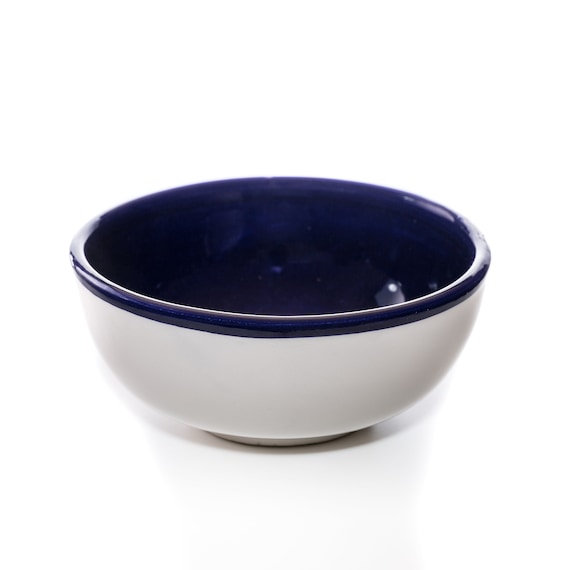The image displays a small to medium-sized, deep ceramic bowl, perfect for serving soup, cereal, or other foods. The bowl features a white exterior that contrasts beautifully with the rich navy blue color lining its interior and the rim. It has a round base and casts a shadow toward the rear, indicating the direction of the light source. The bowl's glossy finish reflects the light along its rim and inside its blue interior, adding a shiny allure to its simple yet functional design. The background and surface are pure white, creating a clean and uncluttered look, likely intended for a catalog or online store.